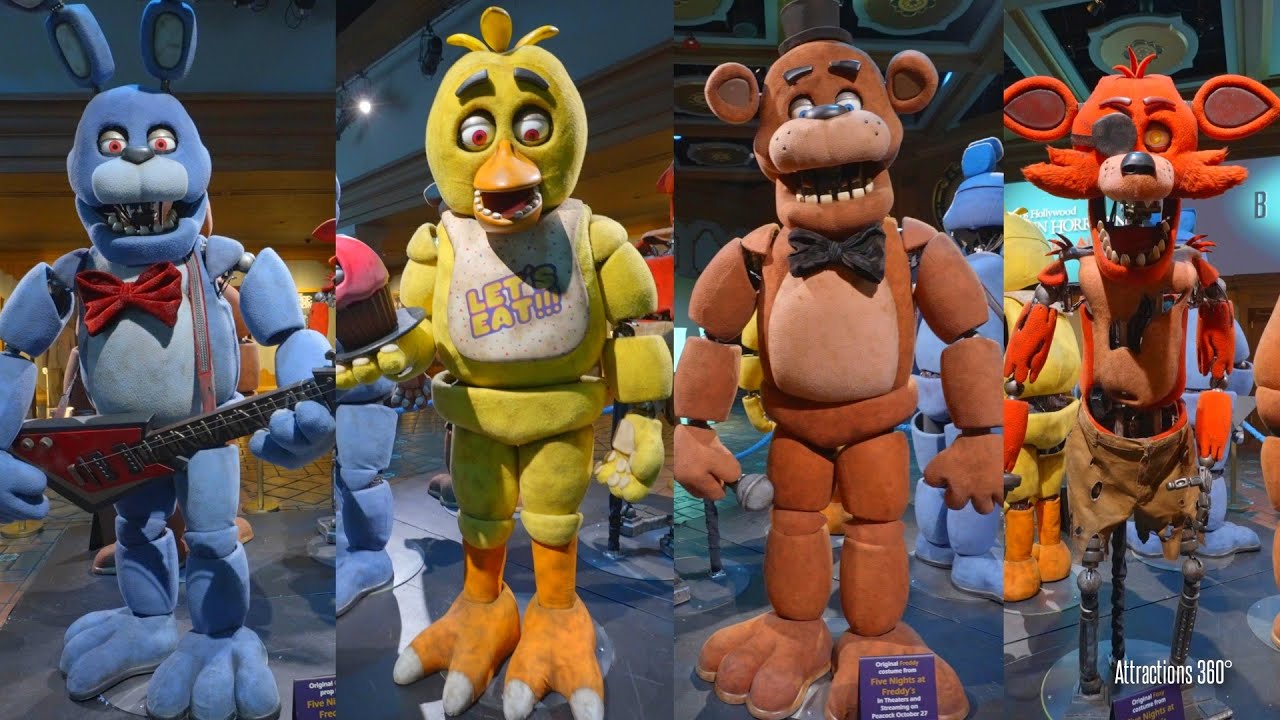This image is a highly detailed photograph featuring four separate animatronic characters from the "Five Nights at Freddy's" franchise, arranged in a rectangular collage. At the bottom right corner, white text reads "Attractions 360 Degrees," suggesting an exhibit or promotional material. Starting from the top left, the first animatronic is a sinister-looking blue bunny with a red bowtie and holding a red electric guitar, with visible mechanical parts. Next to it is a large yellow duck, sporting an orange beak and a white bib that reads "Let's Eat," along with orange feet and white claws. The third character is a brown bear adorned with a black top hat and bowtie, exposing its teeth. Lastly, there is a red fox with an eye patch, wearing tattered brown shorts that reveal its metallic legs. The background includes additional animatronic figures, hinting at a larger display, possibly in a themed venue or a convention setting.